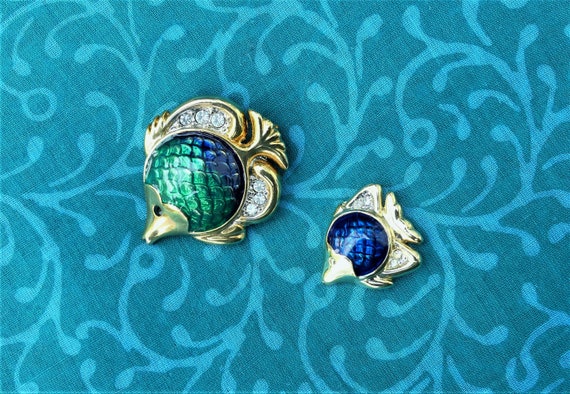This image features two intricately designed brooches or pins set against a medium blue cloth adorned with a lighter blue paisley or tribal-inspired pattern. The focal points are two stylized fish made from gold. The larger fish is embellished with six diamonds—three at the top and three at the bottom—and showcases green and dark blue scales, along with a single black eye. The smaller fish, also gold, features a deep royal blue color with scales and includes two to four diamonds arranged near the top and bottom. The brooches are arranged to emphasize their detailed craftsmanship and vivid colors, beautifully contrasted by the blue patterned fabric backdrop.